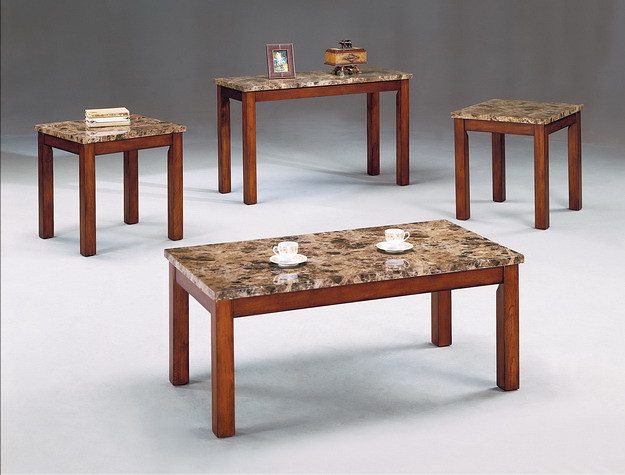This photograph captures an indoor setting showcasing a collection of four matching tables arranged in a neat formation. They stand on a seamless white floor against a grey background, creating a minimalist and spacious atmosphere. Each table features a polished, brown and black speckled marble top with a medium reddish-brown wooden border underneath and matching legs. The front-most table, rectangular in shape, is adorned with two white teacups with saucers. Flanking it are two square, end table-style pieces. The left end table holds a small stack of books, while the right one is unadorned. At the back, another rectangular table, taller than the others, features a framed picture on its left side and a brown and gold object, possibly a lamp, on its right. This setup suggests a typical product arrangement shot, aimed at showcasing the uniform design and functionality of the tables.